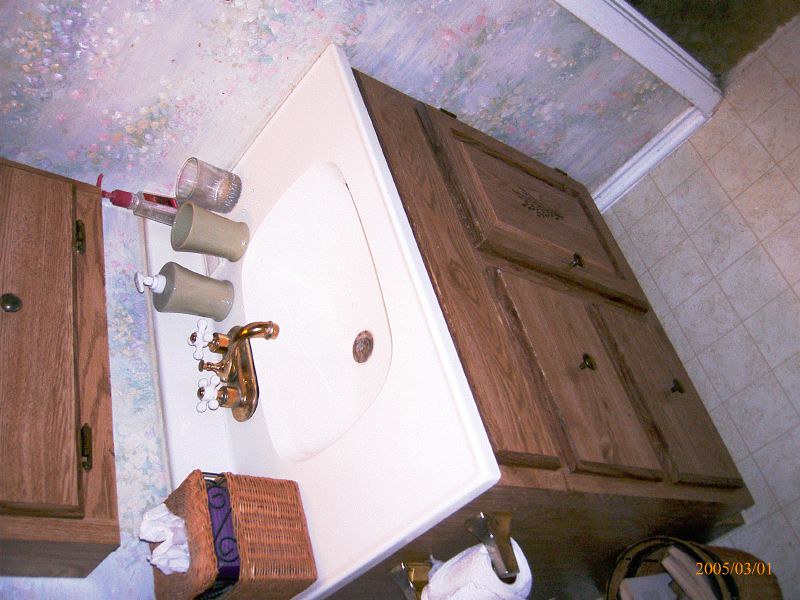A detailed photograph of a bathroom vanity, although tilted 90 degrees to the left, reveals a charming blend of vintage and contemporary design elements. The light gray tile floor is accented with a darker gray trim and medium-sized tiles set with similar color grout. The far wall is adorned with elegant wallpaper featuring a delicate floral pattern in shades of gray and very light, almost pastel green. 

The door trim is a soft off-white color, enhancing the room's subtle palette. Above the vanity is a wooden cabinet with a rich grain, fitted with dark pull knobs and hinges. The cabinet's white top, trimmed with polished brass, complements the vintage-style double-knob faucet with porcelain handles. The sink is seamlessly integrated into the vanity's top, invoking a 1980s or 1990s aesthetic.

To the side of the sink, a wicker basket holds tissues, while a small wastebasket is positioned to the left of the cabinet. The vanity features a single door and two drawers, with a faux drawer front situated behind the sink. This beautifully crafted vanity, dating back to 2005-03-01, showcases a harmonious blend of antique and modern accents.